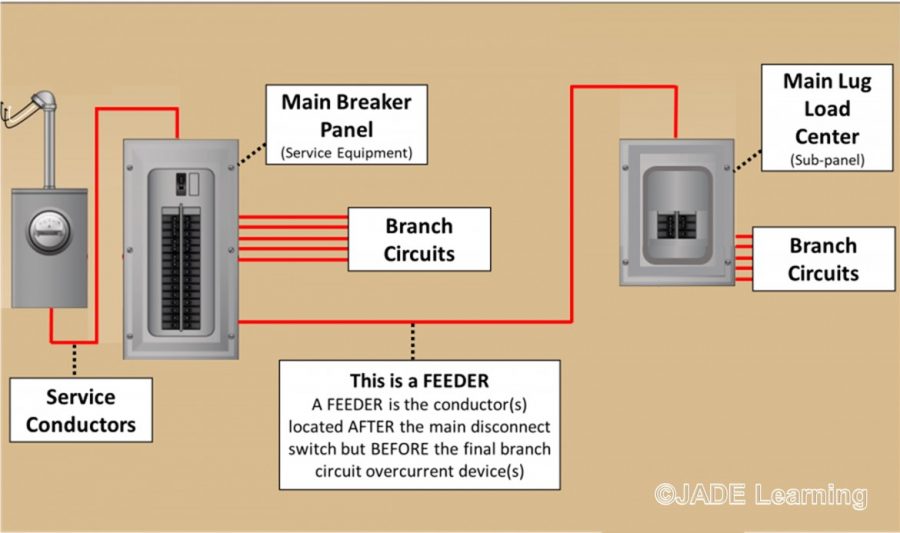The image, which is attributed to Jade Learning, features a detailed diagram against a light tan background, illustrating key components of electrical wiring. The diagram prominently includes several silver-colored, rectangular metal items labeled as service conductors, which are visually connected by red or orange lines indicating the flow of electricity. On the left side, there's a depiction of a main breaker panel serving as the service equipment with black switches housed within a metal border.

The diagram includes white-background labels with black text that identify a variety of electrical components: service conductors, main breaker panel, branch circuits, and a feeder. The feeder, specifically annotated as the conductor situated between the main disconnect switch and the final branch circuit over-current device, is critically highlighted with these red lines for clarity. 

Additionally, there is a main lug load center, also referred to as a sub-panel, shown as a black box with corresponding switches and further connected red lines. All these components are linked, demonstrating the flow and control within an electrical system. Overall, this educational diagram appears less intricate in its color scheme, focusing instead on clearly conveying the relationships and functions of the electrical parts, as intended by Jade Learning.